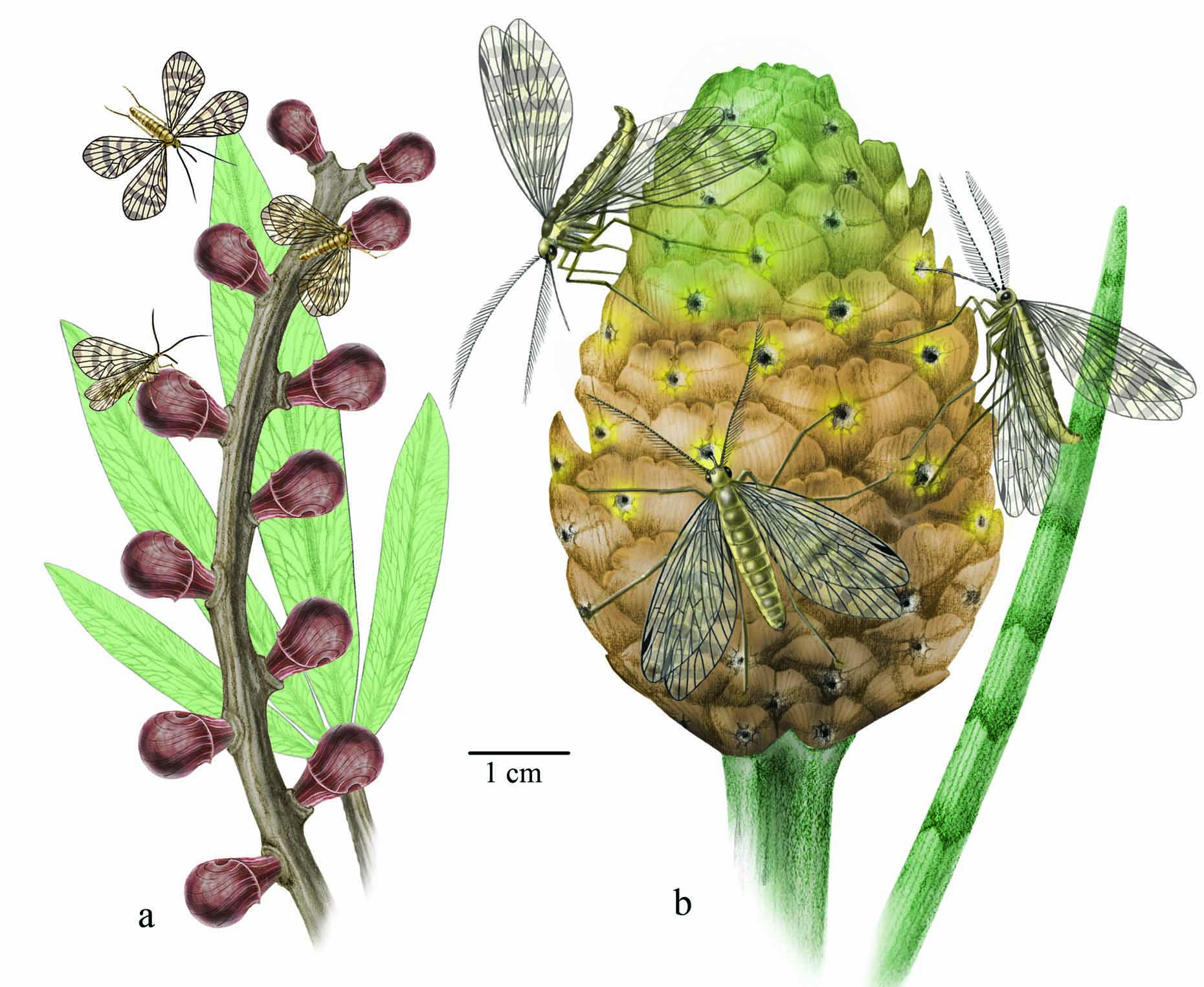In this detailed and animated image, two distinctive plants are depicted with insects hovering above them. The plant on the left features a dark gray stalk adorned with vibrant purple buds that resemble small onions, accompanied by green leaves. Swarming around the buds are what appear to be mosquitoes or possibly tiny wasps. This plant is labeled with a lowercase "a" to its left. 

The plant on the right has a green coloration with a mix of yellow and a conical appearance reminiscent of a pine cone, also populated by similar insects. This plant is marked with a lowercase "b" on its right. Between the two plants, a scale indicator reads "1 cm," highlighting the relative size of the plants. The overall clarity of the image is enhanced by bright natural light, making the colors and details stand out vividly.